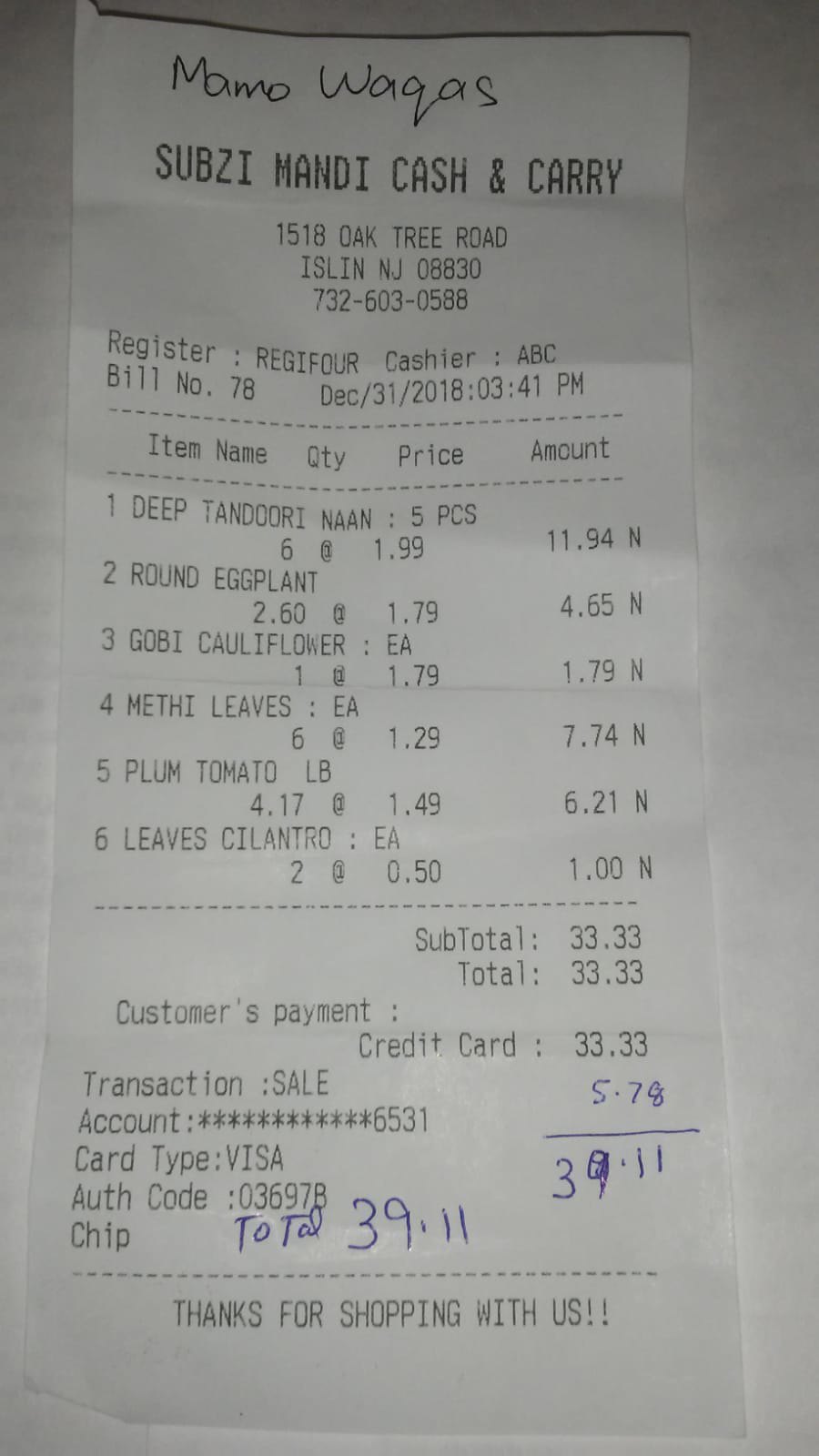This detailed photograph captures a vertically-oriented white receipt from Subzi Mandi Cash and Carry, set against a plain gray background. The receipt is topped with the handwritten text "Mamo Wagus." Below, bold black print displays the store's name, "SUBZI MANDI Cash and Carry," with the address "1518 Oak Tree Road, Iselin, New Jersey 08830," and the phone number "732-603-0588" centered beneath it.

The purchase was processed at Register 4 by cashier ABC, documented on bill number 78. The transaction took place on December 31, 2018, at 3:41 PM. The receipt itemizes the following purchases:

1. Deep Tandoori Naan (5 pieces, 6 at $1.99) totaling $11.94.
2. Round Eggplant ($2.60 at $1.79 per pound) totaling $4.65.
3. Gobi Cauliflower (1 at $1.79 each) totaling $1.79.
4. Methi Leaves (each, 6 at $1.29) totaling $7.74.
5. Plum Tomatoes (4.17 pounds at $1.49 per pound) totaling $6.21.
6. Cilantro Leaves (2 at $0.50 each) totaling $1.00.

The receipt indicates a subtotal and total of $33.33, paid using a Visa credit card. The transaction details include the sale account number 6531, authorization code 036978, and mention of a chip. Handwritten in blue pen beneath the total, additional calculations sum up to $39.11. The receipt concludes with the message "Thanks for shopping with us" in black print.